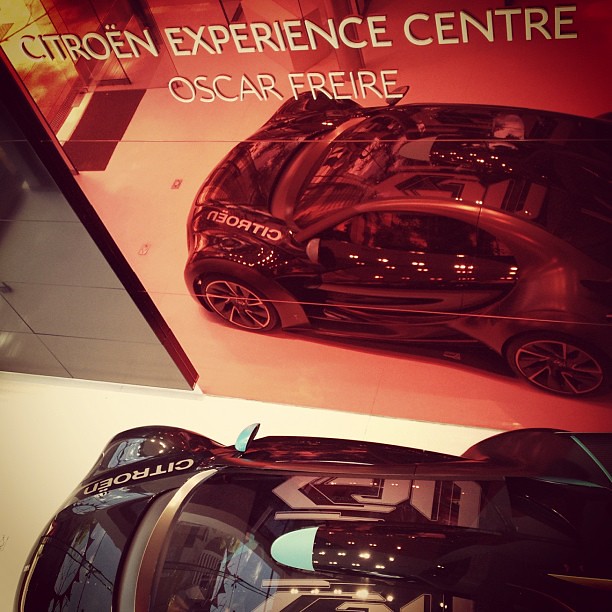The image depicts a striking, glossy black Citroen sports car parked in front of a reflective, polished wall, likely made of an orange metallic or stone material. The polished surface mirrors the car's details, including its sleek roof and sides. Beside this reflective section is a contrasting black stone wall, accentuating the car's bold appearance. On the wall, vivid text reads "Citroen Experience Center, Oskar Freire," which is also inscribed on the car, affirming its association with Citroen. The vehicle features blue accents, notably on the wing mirrors, adding a touch of color to its otherwise black exterior. The ground beneath the car appears white, but the reflection makes it look red, aligning with the polished wall's hue. This detailed interplay of reflection and color gives the image a dynamic and modern feel, highlighting the car's luxurious and high-performance nature.